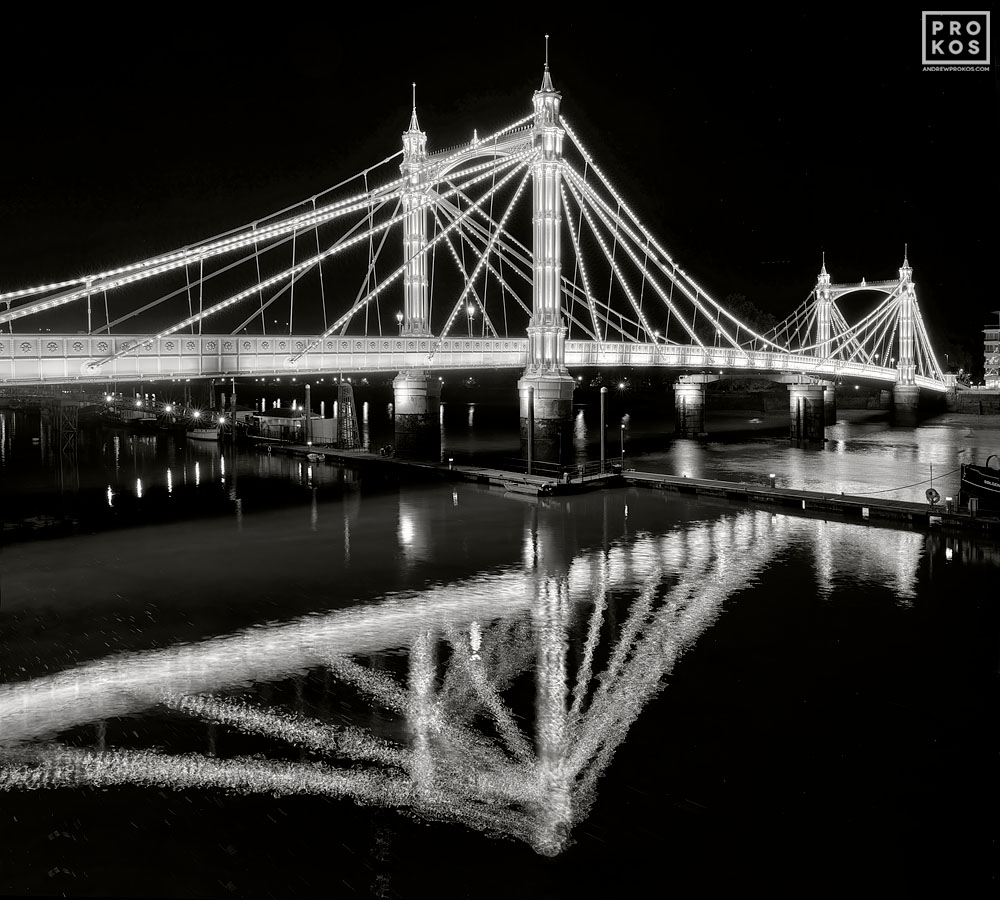This black and white nighttime photograph showcases a large, illuminated bridge spanning over a dark body of water. The bridge is adorned with numerous lights, creating a striking contrast against the pitch-black sky and water. Tower-like columns, evenly spaced and interconnected by visible supporting wires, rise prominently from the bridge, adding to its grandeur. The reflections of the bridge and its lights shimmer vividly on the water's surface below, mirroring the intricate structure and creating a near-perfect reversed image. In the distance, faint city lights can be discerned, enhancing the depth of the scene. A label at the top reads "Prokos," adding a subtle touch of identity to this atmospheric and meticulously detailed composition.